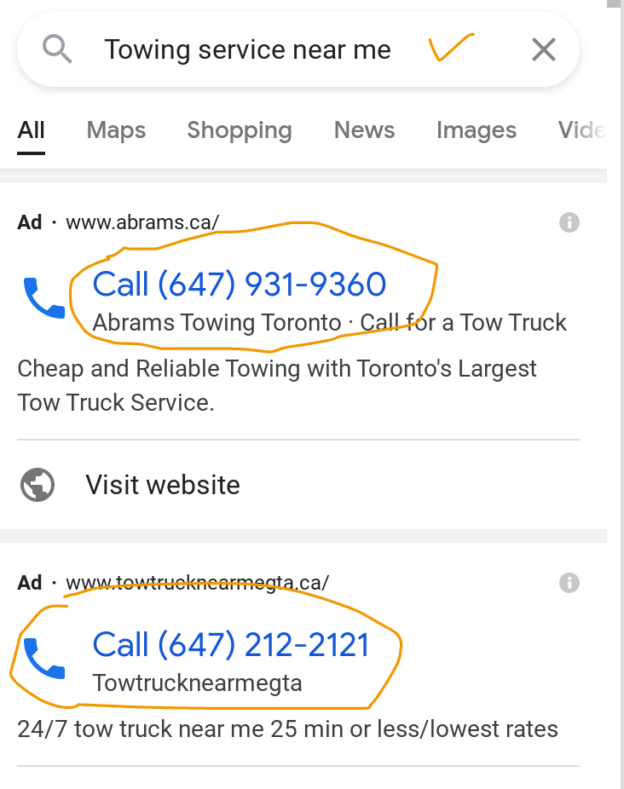This is a detailed screenshot in portrait mode, featuring several handwritten annotations. At the top, a search bar displays the query "towing service near me," with an orange checkmark drawn next to it. Below the search bar, there is a navigation row showing options for various types of results such as All, Maps, Shopping, News, and Images.

The first search result displayed is an advertisement for Abrams Towing, indicated by "abrams.ca" along with a blue clickable link that says "Call 647-931-9360 Abrams Towing Toronto." This link is highlighted with an orange hand-drawn circle around it. Directly under the ad is a "Visit Website" link.

The next line features another advertisement, this one for GTA Towing, with the text "tow truck near me gta.ca" and a phone number "Call 647-212-2121." This phone number is prominently encircled with an orange hand-drawn circle as well.

The annotations suggest that the screenshot is meant to be shared with someone seeking immediate towing services. The orange circles emphasize two local Toronto-based towing service phone numbers, possibly intended to assist someone whose vehicle is currently disabled.